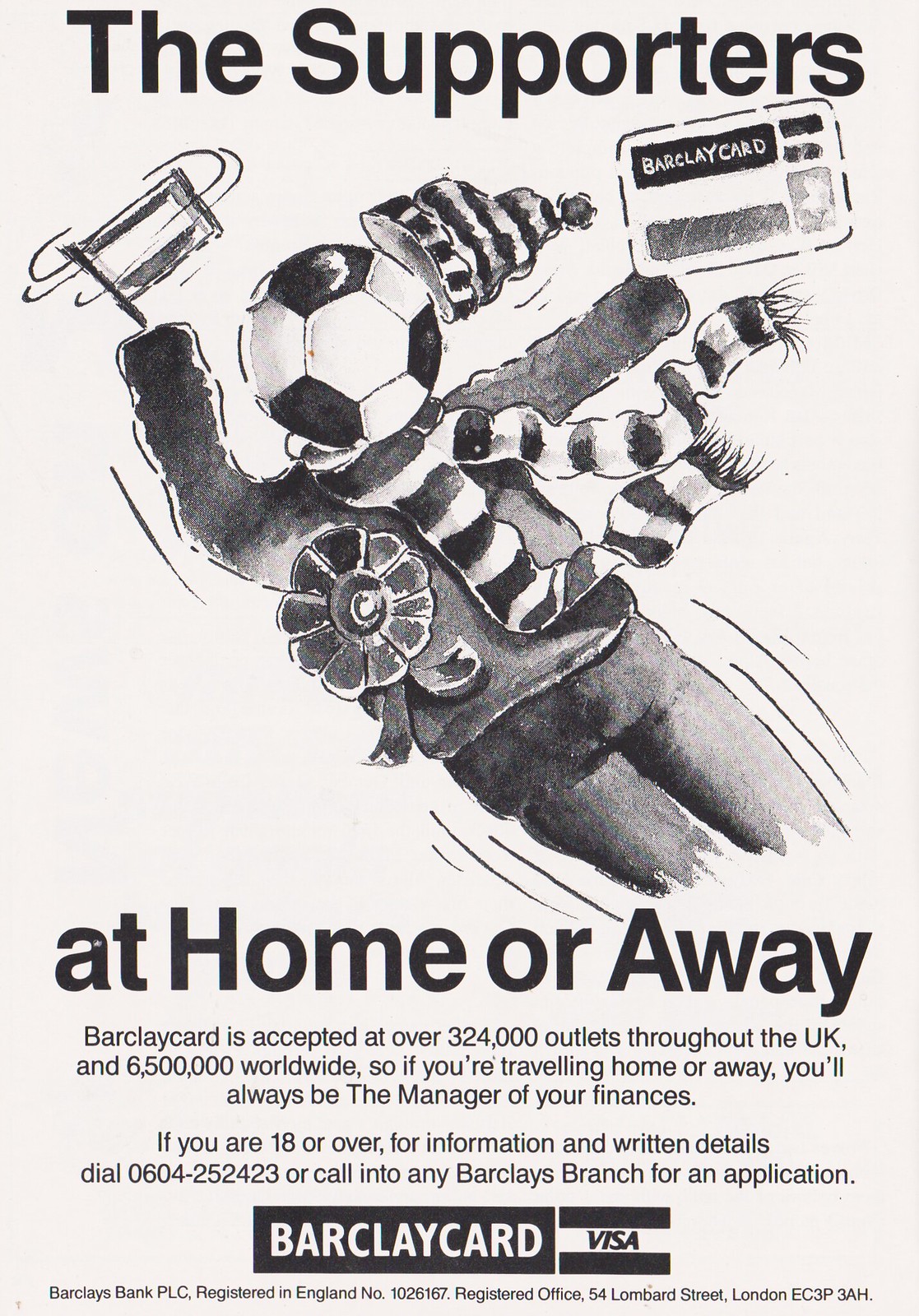This vintage-style Barclaycard advertisement, set against a light grayish background, prominently features the bold heading "The Supporters" at the top. Beneath this heading occupies a major portion of the poster an illustrated humanoid figure with a soccer ball as its head, adorned with a winter ski cap. The figure is dressed in cold-weather clothing that includes a gray-black sweater, a scarf, and pants. A large, flower-petal-shaped ribbon is pinned to the left side of its chest. One of its hands holds a flag, while the other extends a Barclaycard, depicted with detailed designs. The figure appears to be in motion, suggested by dynamic lines around it. Below the illustration, the text "At home or away" is printed in bold, dark black fonts. Further down, the advertisement highlights that Barclaycard is accepted at over 324,000 outlets throughout the UK and 6.5 million worldwide, emphasizing its utility for managing finances both domestically and abroad. The poster includes a contact number, 0604-252-423, for those 18 or over seeking more information or application details, pointing to both a phone line and any Barclay branch. At the bottom center are the Barclaycard and Visa logos, and the footer reads: "Barclays Bank PLC, registered in England, number 1026167, registered office 54 Lombard Street, London EC3P 3AH."